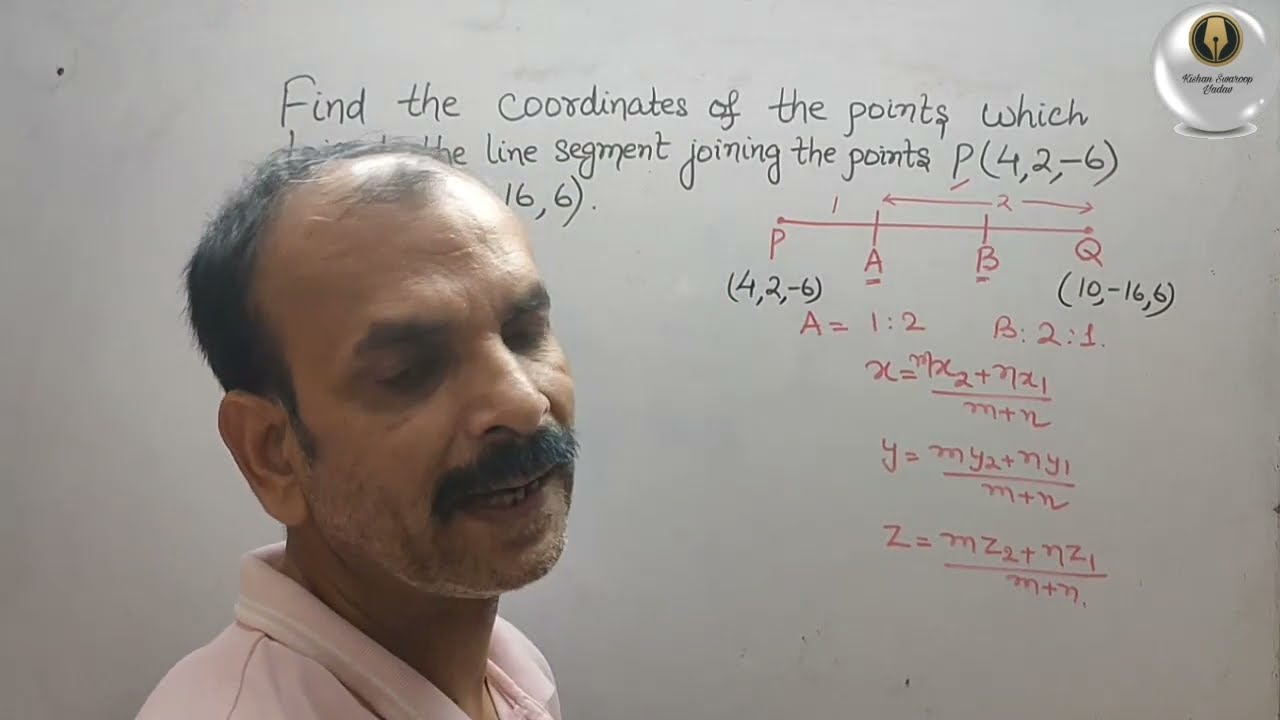In the image, we see a middle-aged Indian man with tan skin standing in front of a stained whiteboard. He is wearing a pink, short-sleeved polo shirt. The man has a thick black mustache, black eyebrows, and a beard area with some gray stubble. He is balding on the front part of his head, but has black hair with some gray patches behind the bald spot, extending to black sideburns. His eyes are closed and the image is cropped at his shoulders.

The whiteboard behind him contains a partially obscured mathematical problem. At the top of the board, it reads, "Find the coordinates of the points," but some text is blocked by his head. Below this, in black font, it states, "line segment joining the points P (4, 2, -6)" followed by "16, 6." There's a diagram in red with a line marked at ends 'P' and 'Q' and intermediate points labeled 'A' and 'B'. The coordinates for P are clearly visible as (4, 2, -6), while those for Q are (10, -16, 6). Additionally, it includes the ratios "A = 1:2" and "B = 2:1." Below these, multiple equations with various variables are displayed, illustrating the steps to solve the problem.